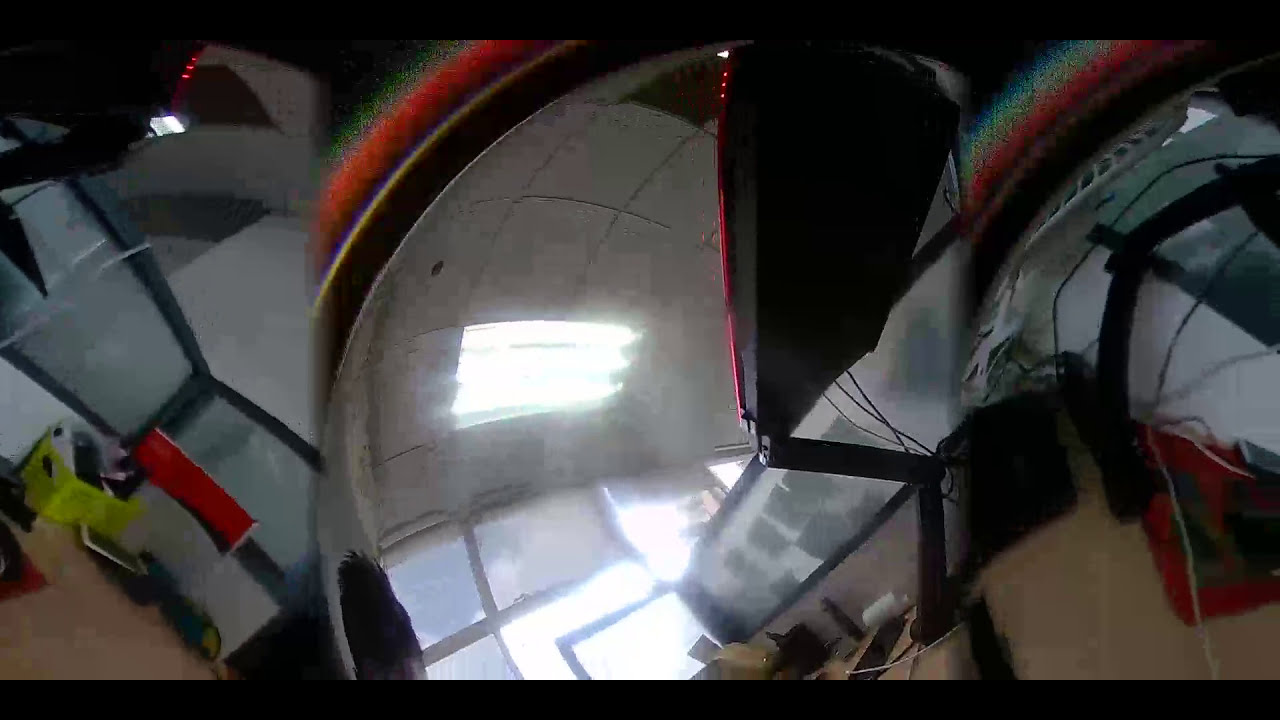The image depicts a cluttered indoor setting with a composite, VR-like, fisheye perspective, giving it a 3D, immersive feel. Central to the image is a ceiling light amidst a congestion of objects, including mechanical equipment with wires, multiple monitors, and desktop items. The scene appears to be a commercial storage facility or office space, characterized by several reflective elements and slanted, curved features suggesting a virtual reality environment. The split, composite image reveals three segments, reflecting off a round lens or fisheye mirror, showing the same room from different angles with a focus on a window with scattered papers and a partial see-through partition separating cubicles. The colors visible are black, brown, red, yellow, blue, green, white, and gray, and the image lacks any textual elements. Overall, the central and prominent objects are the ceiling light, the window, and reflective surfaces providing a chaotic yet detailed glimpse into this indoor space.